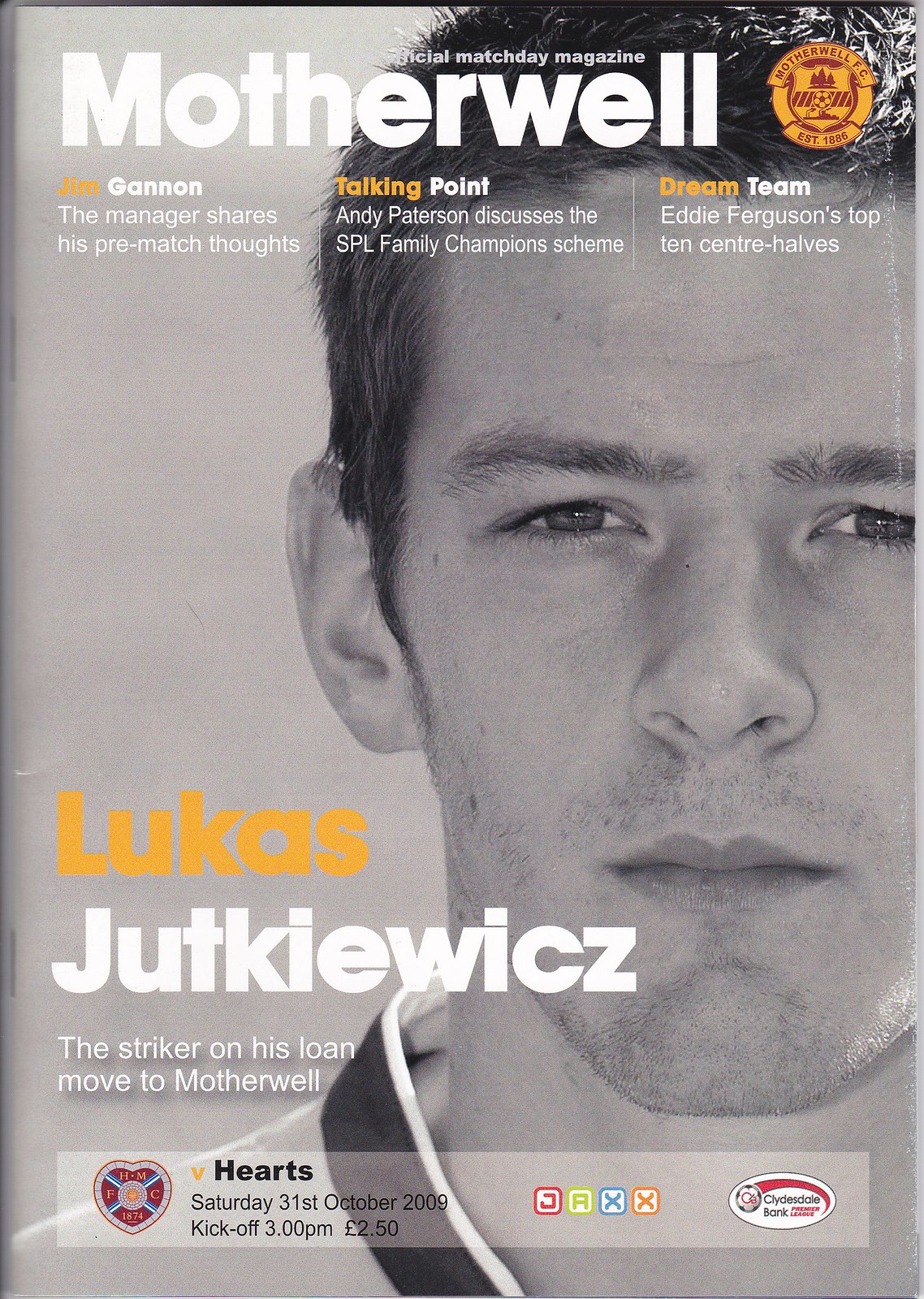This is the cover of the official Match Day Magazine for the professional European football team, Motherwell. The headline at the top features "Motherwell" in large, bold white letters. Below it, a gold logo displays "Motherwell LLC." Dominating the cover is a grayscale photograph of a soccer player with short dark hair and a stern expression, identified as Lucas Jutkiewicz. His name is prominently displayed to the left of his face, with "Lucas" in yellow and "Jutkiewicz" in white. A subtitle beneath his name reads, "The striker on his lone move to Motherwell." Additionally, this issue includes various articles such as the manager Jim Gannon sharing his pre-match thoughts, Andy Patterson discussing the SPL Family Champion Scheme, and Eddie Ferguson's Top 10 Center Halves. At the bottom of the cover, details of an upcoming match are provided, including a small banner in lighter gray that mentions "Hearts" with relevant symbols and the match details: "Saturday 31st October 2009, kickoff 3 p.m."